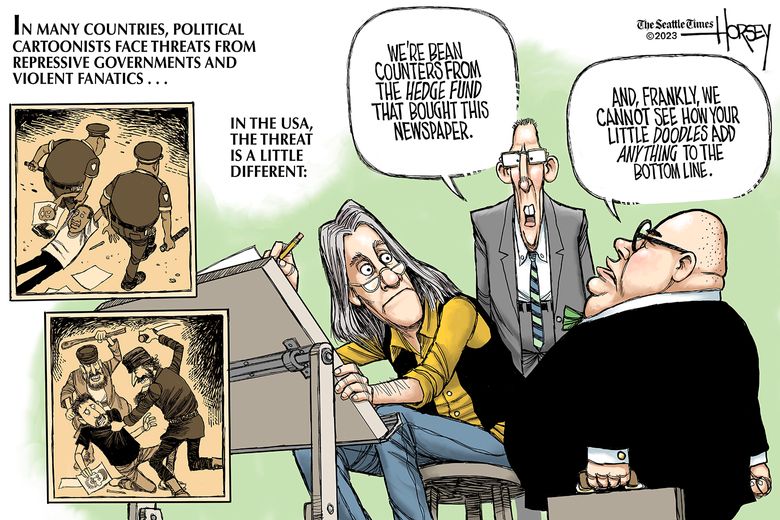This detailed political cartoon, featured in the Seattle Times in 2023 and signed by Horsey, critiques the challenges faced by political cartoonists. The central image depicts a cartoonist at an easel, diligently drawing, while being scrutinized by two businessmen. One, a gaunt figure in a gray suit, declares, "We're bean counters from the hedge fund that bought this newspaper," to which his portly colleague in a black suit and glasses adds, "And frankly, we cannot see how your little doodles add anything to the bottom line." Surrounding this main scene are smaller vignettes highlighting the global plight of cartoonists. In one corner, a harrowing scene shows two police officers violently beating a cartoonist, with a caption stating, "In many countries, political cartoonists face threats from repressive governments and violent fanatics." Another box portrays a cartoonist being dragged away by armed guards. Through this juxtaposition, the cartoon underscores the different, yet serious, threats to artistic expression both internationally and within the United States.